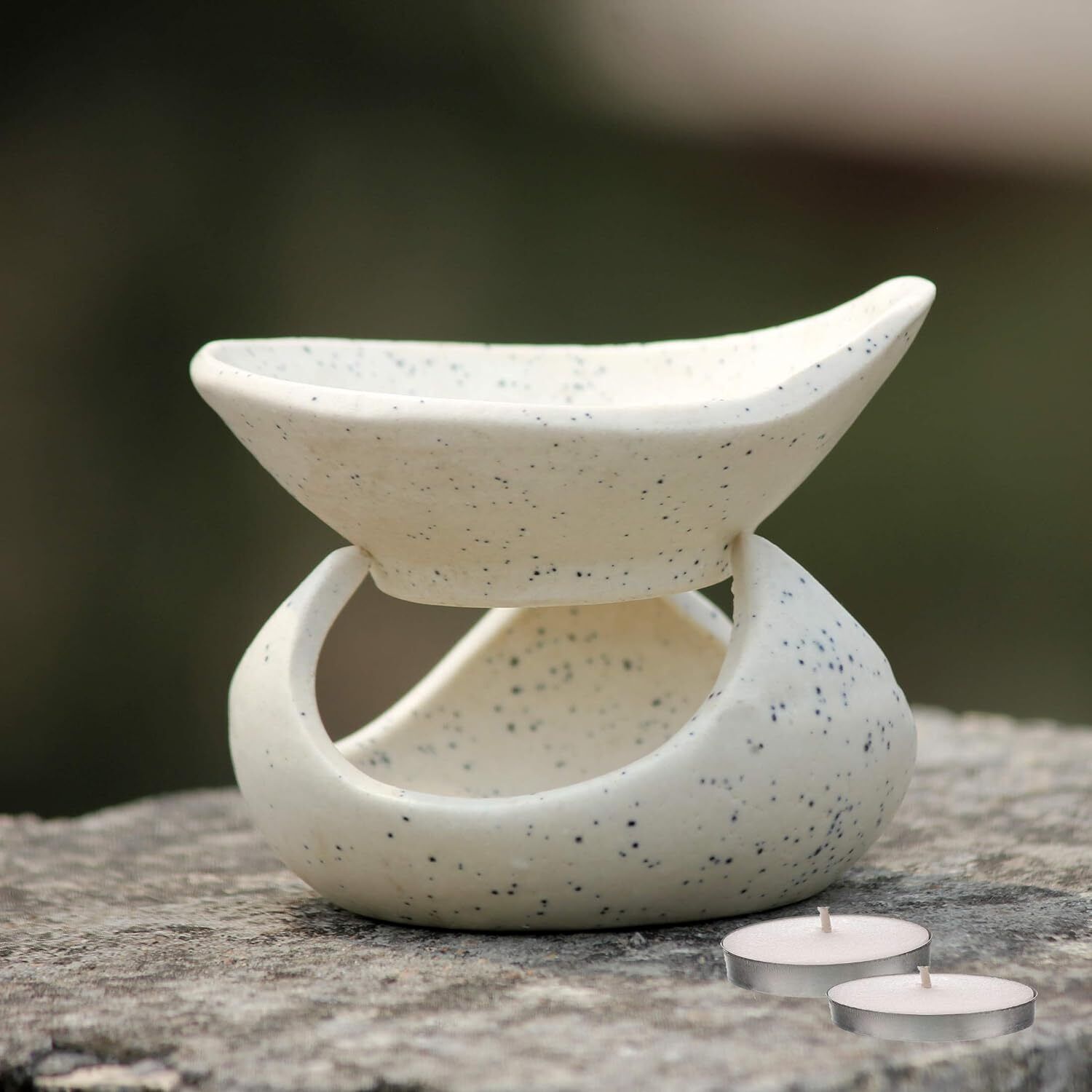This realistic, square-shaped photograph appears to be taken outdoors, given the green and blurry background. At the center of the image is a unique, two-tiered sculpture, predominantly white with specks of blue or black, resembling either a decorative piece or white chocolate. The bottom section of the sculpture has three rounded, upward-curving points that form a triangular base, supporting an oval-shaped bowl on top. Adjacent to the sculpture are two small, disc-shaped tea light candles. These candles are white with short wicks, encased in gray or silver holders and are about the size of a thick silver dollar. The sculpture and candles are set upon what looks like a wooden table.